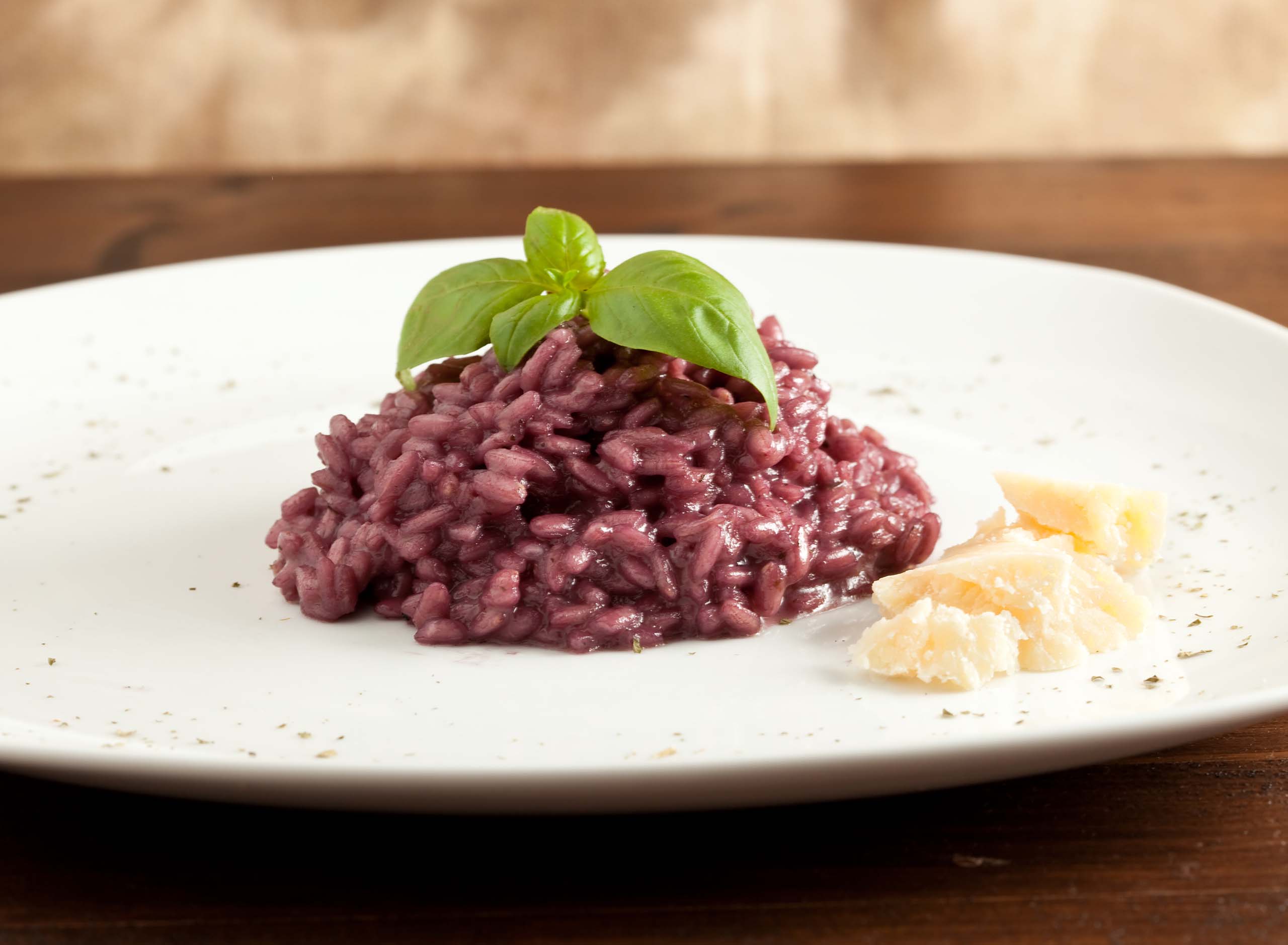This image features a round, white ceramic plate resting on a dark-finished wooden tabletop. The background reveals part of a brownish-white wall. At the center of the plate is a small mound of purple or burgundy-colored rice, possibly cooked with red wine, giving it a rich, unique hue. The rice is accompanied by a small mint leaf or fresh basil sprig on top for garnish. To the right of the rice, there are crumbles of a dry, crumbly cheese, such as manchego or parmesan. The plate is adorned with a light sprinkle of purplish specks, possibly herbs or a decorative drizzle, enhancing the overall aesthetic of the dish.